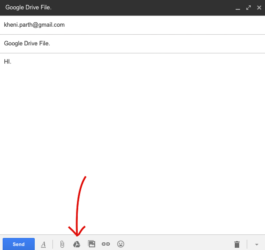The image appears to be a screenshot of a Google Drive file interface. At the top of the image, there is a black navigation bar extending horizontally across the screen. On the left side of this black strip, the text "Google Drive File" is prominently displayed in white font. To the right side of the strip, there are three small icons: a dash or underscore, a diagonal arrow, and an "X." 

Below the navigation bar, the background turns white. In black letters, an email address is partially visible, appearing to be "carryparty@gmail.com" or something similar, though it is slightly blurry. Further inspection reveals a partially legible username, likely "KHE..." possibly followed by "N I" or "R I," though this too is difficult to decipher clearly.

A thin gray line is positioned below the email information, followed by the text "Google Drive File" once again. Another gray line separates this text from additional content below it. The next visible content is slightly blurry, but it appears to start with a capital "H" and could be part of a sentence or a heading.

At the very bottom of the image, there is a gray strip. On its left side, a small blue rectangle is situated with the word "Send" displayed in white. Adjacent to this blue rectangle are several small icons or images. The third icon closely resembles a recycling symbol, and a red arrow is directed towards this specific symbol, pointing downward.

Overall, the image showcases a typical view of a Google Drive file with various navigational and functional elements.